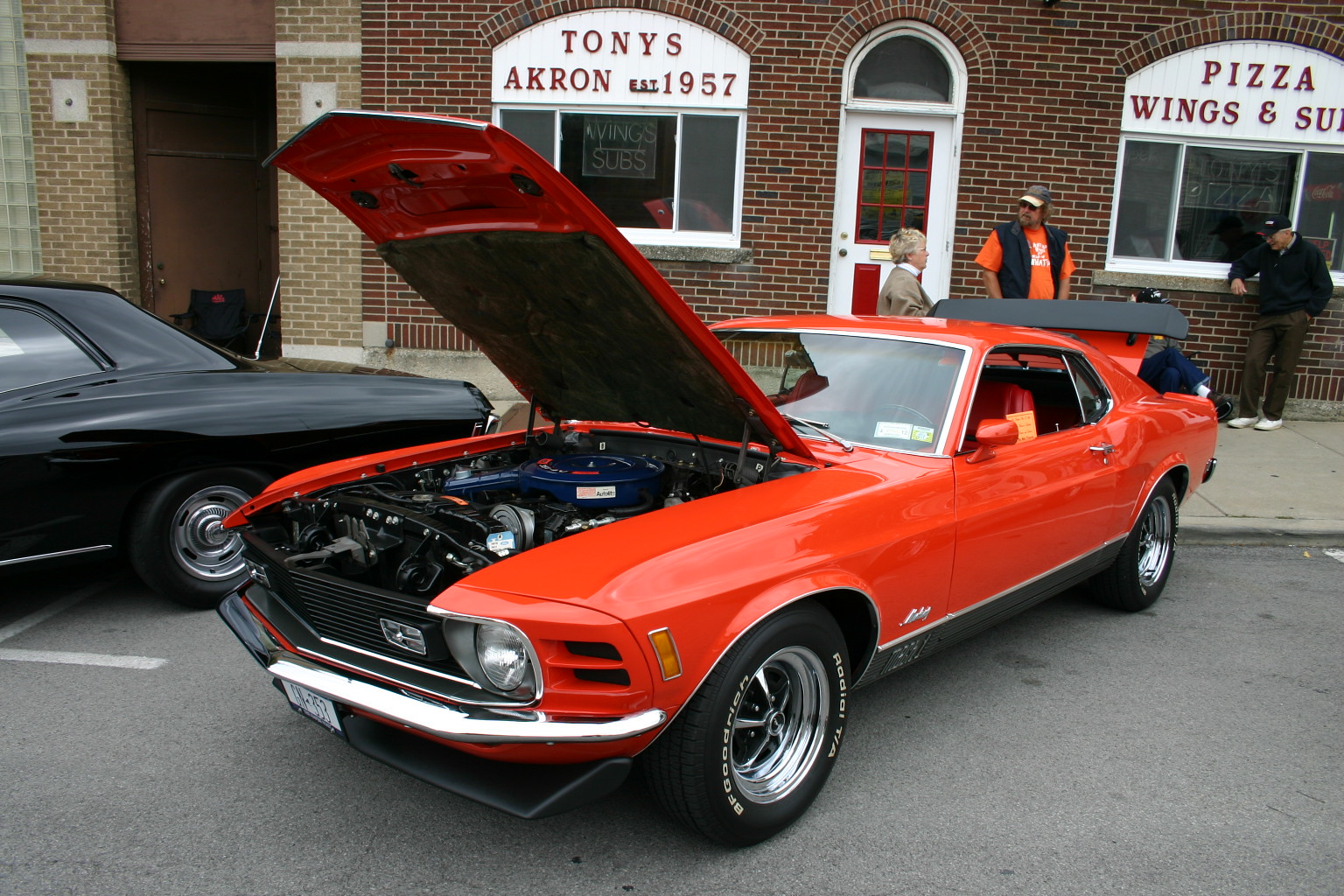In the image, we see a detailed, outdoor scene centered around a vibrant orange car displayed at a car show on an asphalt road. The car sits directly in the middle of the photo, angled diagonally with its hood open to reveal a meticulously clean motor, showcasing features like the carburetor. It has sleek silver rims and black tires, and the windows and trunk are also open. To the left, the rear portion of a shiny black car is partially visible, displaying a hint of its polished body and windows.

In the background, a red-brick building with tan accents provides a backdrop. The building is marked with a large sign in bold red letters that reads "Tony's, Akron 1957" and advertises "Pizza, Wings, and Subs." The setting appears to be a parking lot in front of this sub shop, suggesting a mid-day car display event. Several people are seen standing on the sidewalk, engaged in conversations, adding a lively atmosphere to the scene. The colors prominent in the image include shades of gray, white, red, orange, black, blue, brown, and tan, contributing to a visually vibrant and dynamic composition.